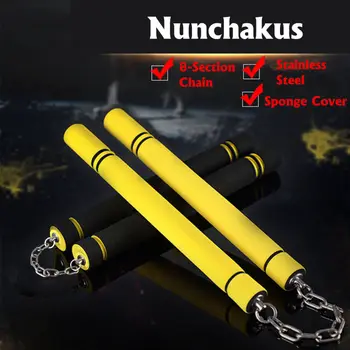The image displays two pairs of nunchakus set against a predominantly dark background with a gray area resembling a table surface at the far end. The top pair of nunchakus is bright yellow with black rings—two at the top and one at the bottom—connected by a silver metal chain. Below them is another pair of nunchakus, which are black with yellow rings—similarly arranged with two at the top and one at the bottom—and also connected by a silver metal chain. In the top right corner of the image, the word "Nunchakus" appears in white text. Below this, a checklist written in red font is displayed, detailing features such as "A-section chain," "stainless steel," and "sponge cover," each accompanied by a red check mark. The overall scene is dominated by the contrast between the nunchakus' striking colors and the dark backdrop.